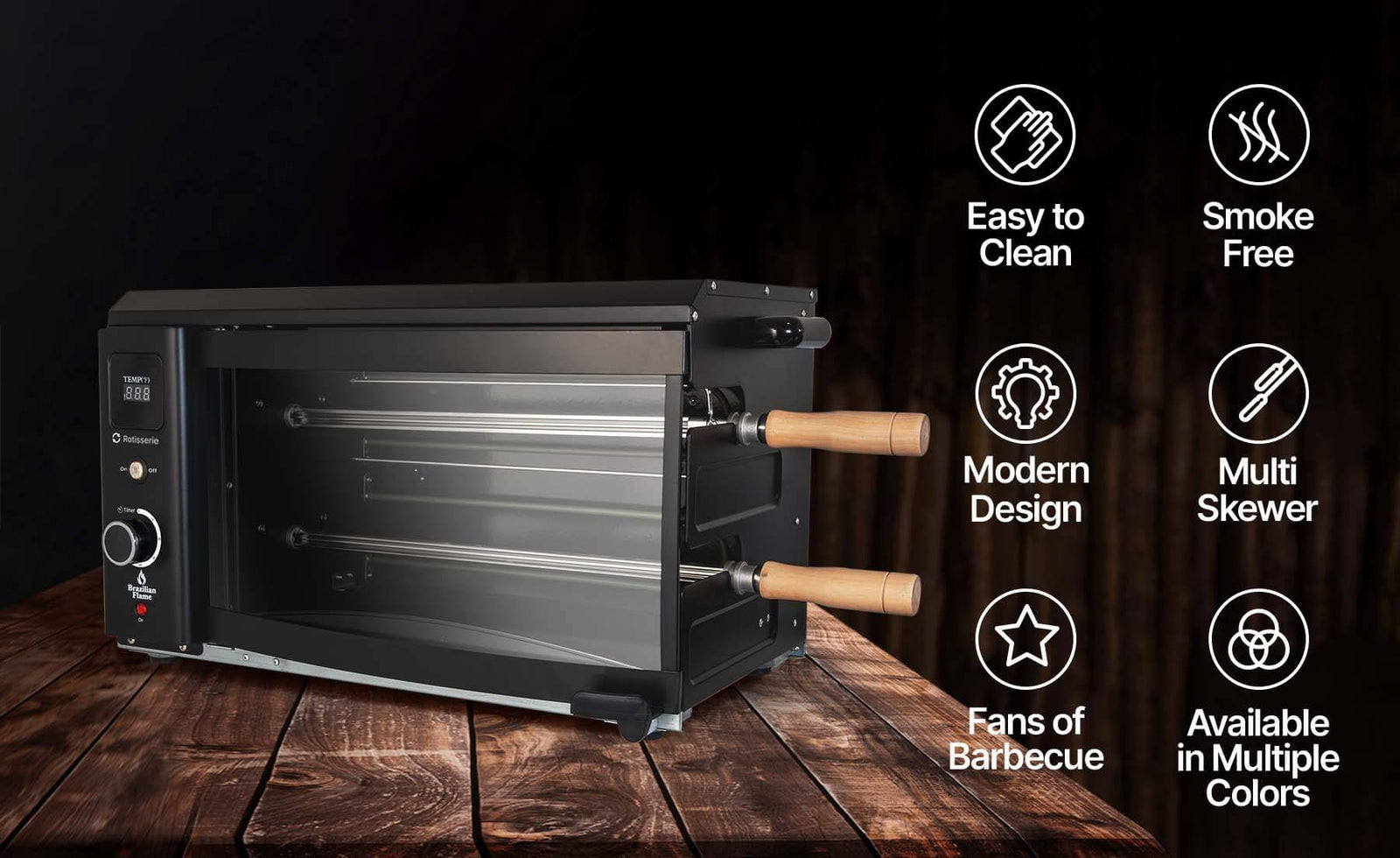The image is an advertisement for a compact, personal-sized rotisserie oven, designed for barbecue enthusiasts. This sleek, modern oven features a flat matte black finish typical of high-end barbecues. It is placed on a rustic wooden table, resembling a picnic bench. The oven is equipped with two long, thin silver skewers with wooden handles that extend out of the machine, ideal for cooking multiple items like chicken simultaneously. The oven includes a glass front and a single temperature control knob on the left side with a white rim. On the right-hand side of the image, there are several white-outlined graphics and text, highlighting key features: easy to clean, smoke-free, modern design, multi-skewer functionality, designed for fans of barbecue, and availability in multiple colors. Overall, the well-designed oven promises both functionality and ease of use, making it an attractive tool for versatile barbecue cooking.